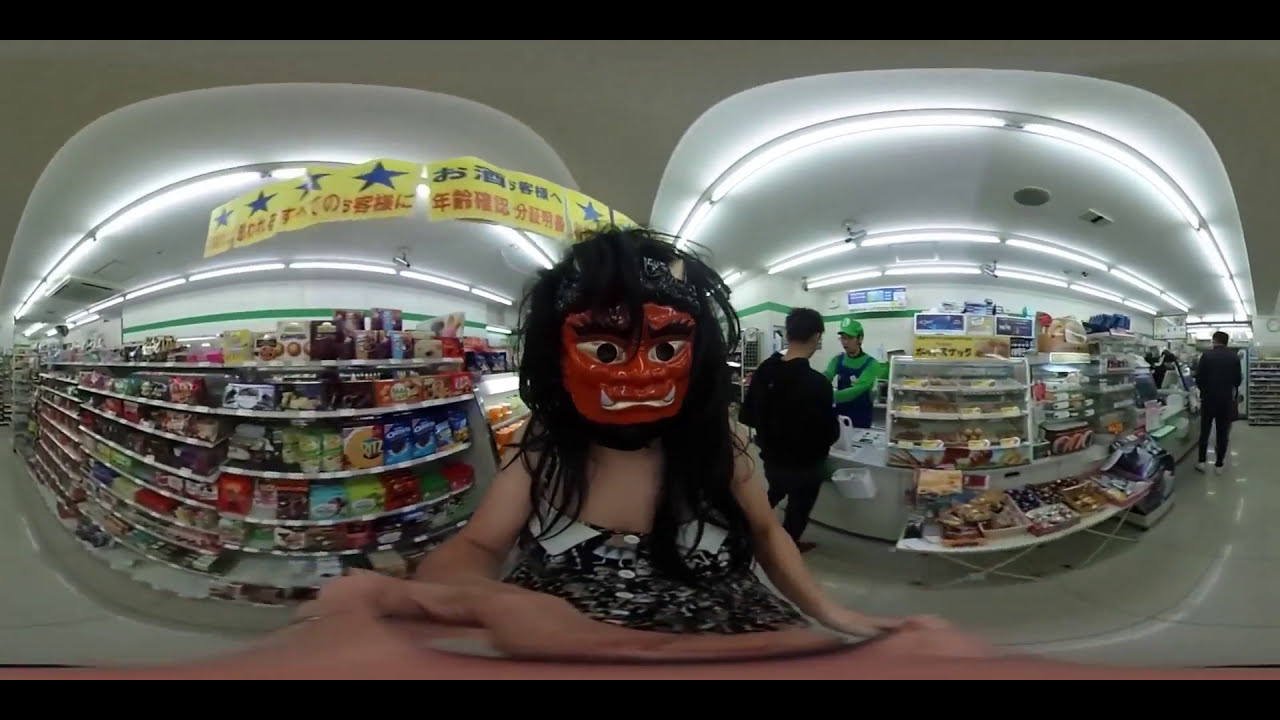This is a 360-degree panoramic photograph set in a shopping mall, specifically at a deli or pharmacy counter. The central figure is a woman with long black hair, dressed in a black and white patterned dress, and wearing a vivid red demon mask complete with horns and fangs. This striking mask gives her an eerie, sinister appearance. The surrounding scene reveals extensive details: shelves stocked with snacks, including Oreo cookies and Ritz crackers, span both sides of the image with LED tube lights illuminating the white ceiling. A yellow banner adorned with red letters and blue stars hangs prominently from the ceiling. To the left, a detailed view of the shelves reveals various packages across seven rows, while a display case sits on a counter nearby. Further to the left, a person is visible waiting as another individual pays for their goods at a prop-open table in front of the display case. On the right side, another man stands near a counter, and a person can be vaguely seen behind this counter, all contributing to the bustling yet surreal atmosphere captured in the photograph.